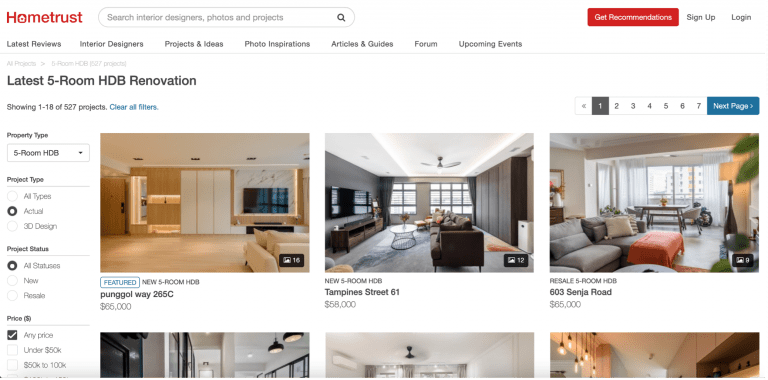Screenshot of the Home Trust website displaying interior design projects and their costs. The interface has a clean white background. In the upper left corner, the red text "Home Trust" is prominently displayed. Adjacent to it is a search bar that reads "Search Interior Designs, Photos and Projects." On the right-hand side, there's a red button labeled "Get Recommendations."

Navigational tabs run across the middle of the page, offering categories such as "Latest Reviews," "Interior Designers," "Projects and Ideas," "Photo Inspirations," "Articles and Guides," "Forum," and "Upcoming Events." Below, a headline in black text announces "Latest 5-Room HDB Renovation."

The section showcases six images, although only the first row of three is fully visible, with the second row partially cut off. 
1. The first image depicts a living room setup that appears to be in progress, captioned "Featured 5-Room HDB with a cost of $66,000."
2. The second image shows another living room with a series of windows along the back wall and is labeled "Tampines Street, $61,000, $58,000."
3. The third image features a living room with a gray sofa and a similar row of windows, titled "$65,000 at 603 Sandra Road."

Above the images, navigational indicators show the current page as "1 of 7," with page number one highlighted in black.